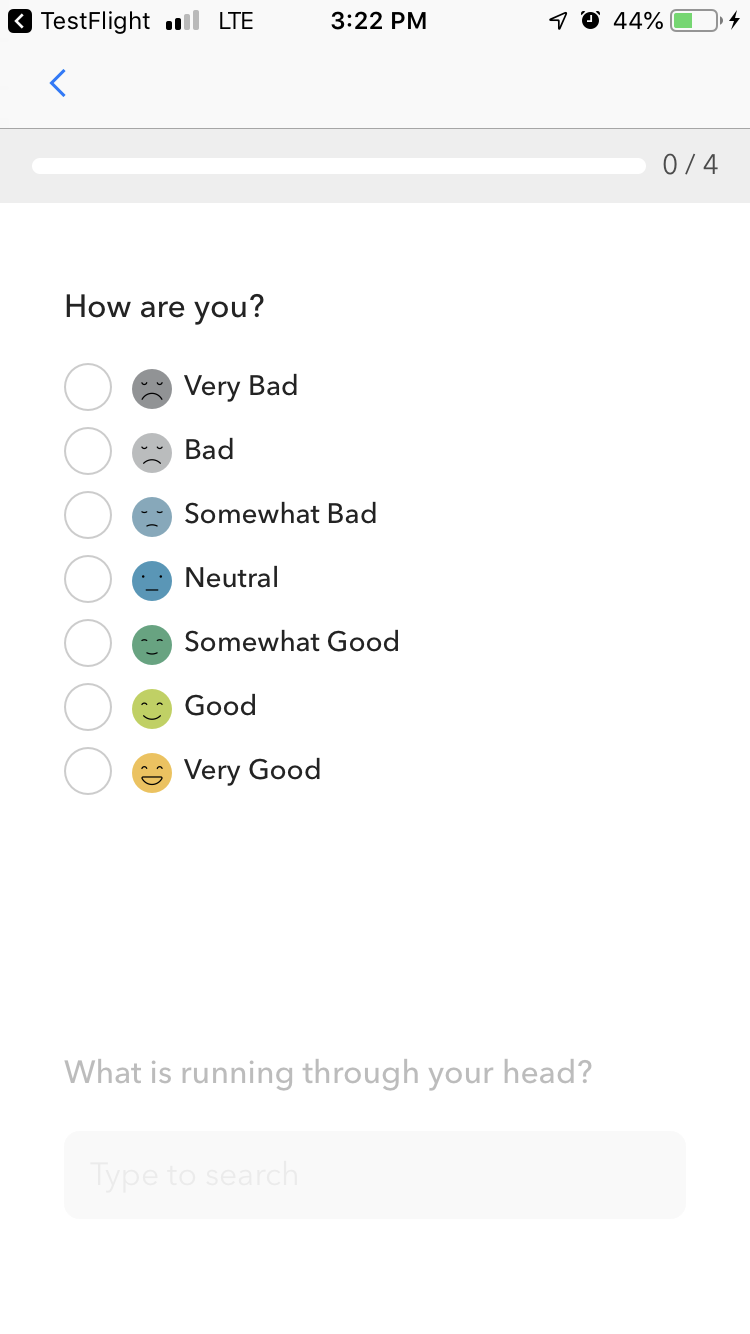Caption:
A visual interface from a test flight is displayed at 3:22 PM, showing key telemetry details. The LTE signal strength is noted as two out of four bars, while the battery level is at 44%, indicated by a green battery icon with a lightning bolt. A user interface element, consisting of blue arrows and a white bar on a gray background, shows "0/4."

Additionally, a feedback mechanism showcases various emotions through icons. These range from a circle with a sad face indicating "very bad," progressively changing to a circle with a large grin representing "very good." The interface prompts users with a "What is running through your head?" input field, accompanied by a "Type to search" prompt.